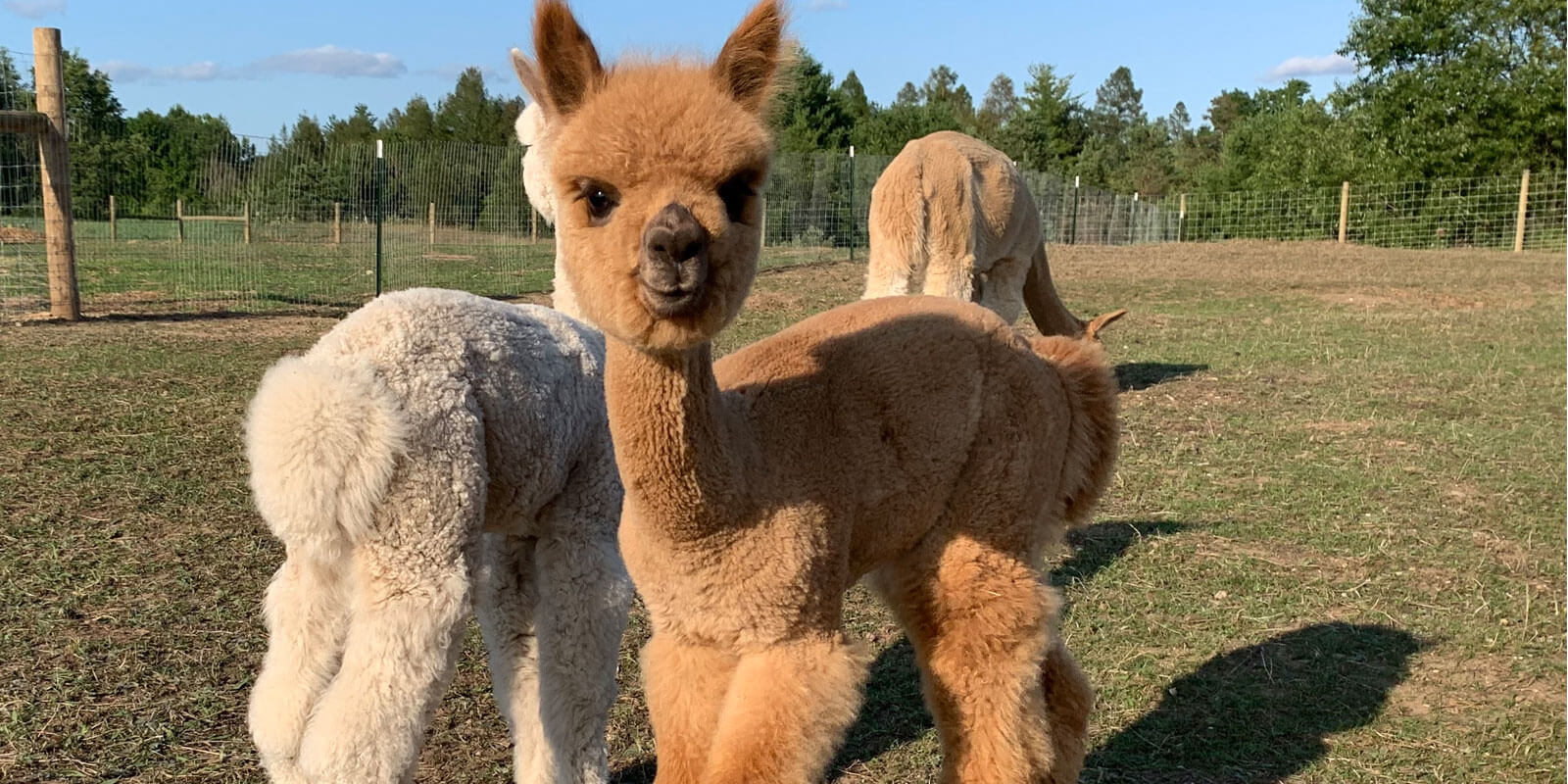In this vibrant outdoor photograph set in Peru, three freshly groomed alpacas, two tan and one beige, stand prominently in the center of a grassy field. The alpacas are positioned such that one looks to the left, another faces the right, and the third has its back towards the camera, creating a dynamic composition. A rustic wicker fence with wooden stakes runs behind them, leading the eye to a vivid treeline at the back of the scene. The field itself is a mix of green and dead yellow-brown grasses, while the clear blue sky overhead enriches the pastoral setting under the daylight.